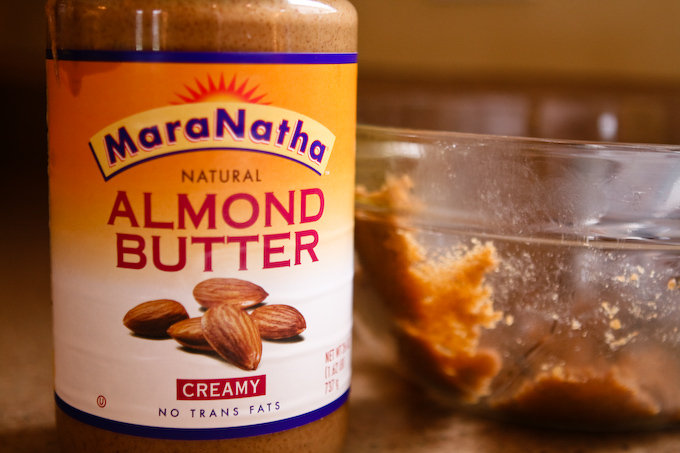This close-up image depicts a jar of MaraNatha brand almond butter. The jar's label features a distinctive design, starting with an orange banner that fades into white, with blue borders. At the top, the yellowish banner has blue text outlined in red that reads "MaraNatha," with the sun's rays peeking above it. Beneath this header, in blue text, it states "natural" followed by bold red capital letters reading "ALMOND BUTTER." The label also includes an image of almonds. Below that, in a red rectangle, the text "creamy" is displayed, with "NO TRANS FATS" written in small caps at the bottom. Positioned to the right of the jar is a clear bowl containing visible bits of almond butter, all set against a brown wooden surface. The background is unobtrusive, devoid of any distracting elements, drawing full attention to the almond butter jar and bowl.